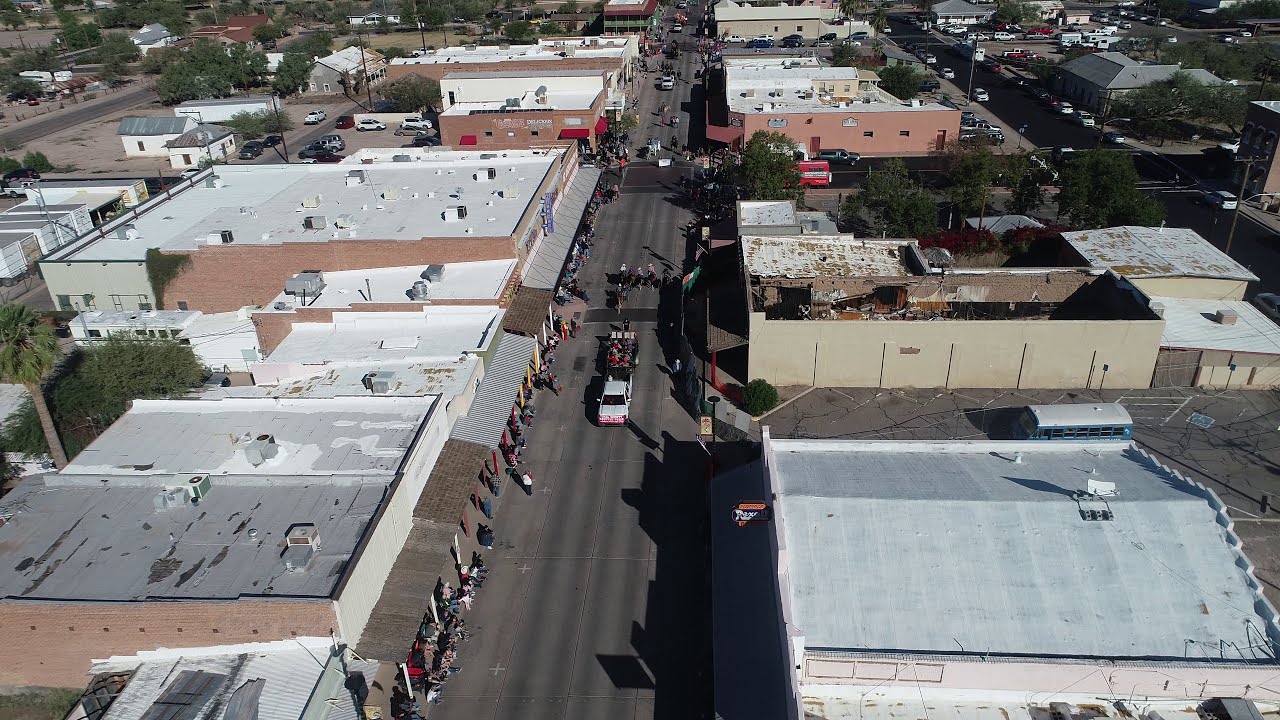This vibrant and detailed aerial photograph captures the essence of a bustling town on a bright, sunny day. Central to the image is a straight, grey main street running vertically from the top to the bottom, adorned with vehicles and spectators, suggesting a parade in progress. The street is flanked by one- and two-story buildings, their close proximity casting noticeable shadows onto the road. The architectural variety includes flat and conical roofs, painted in shades of white, tan, brown, and a striking light blue.

On either side of the parade route, people can be seen lining the sidewalks, adding to the festive atmosphere. Various vehicles, including trucks and possibly motorcycles, are staggered along the street, reinforcing the parade theme. In the distance, the landscape transitions to smaller houses interspersed with trees and greenery, breaking the dense pattern of the town center. To the far right, a blacktop road suggests additional traffic flow.

The scene is bathed in midday sunlight, as evidenced by the shadows directly beneath the buildings, highlighting the vibrant colors and the dynamic activity of the small city. Overall, this image beautifully captures an engaging moment, combining architectural details with the lively human element of a community gathering.